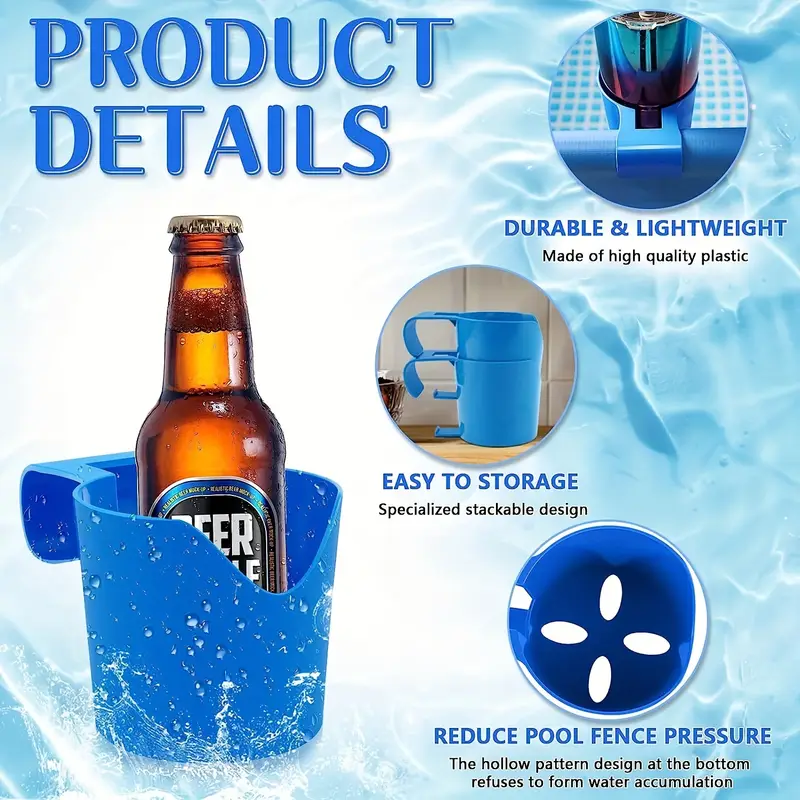This promotional image has a blue backdrop that mimics a water surface, evoking the setting of a swimming pool. At the upper left corner, it says "Product Details" in blue text. Dominating the left side of the image is a detailed rendering of the product – a blue drink holder designed for above-ground pools. The holder, shown with a glass beer bottle inside, features a clip that securely attaches to the pool's edge, ensuring beverages don't end up in the water.

On the right side of the image, three blue circles sequentially highlight the product's benefits. The top circle states "Durable and Lightweight, made of high-quality plastic," emphasizing the robustness and ease of use. The middle circle mentions "Easy to Store, Specialized Stackable Design," illustrating how the drink holders can nest inside each other for compact storage. The bottom circle notes "Reduces Pool Fence Pressure, the hollow pattern design at the bottom prevents water accumulation," explaining how its thoughtful design minimizes stress on pool fences and avoids water build-up.

Additionally, another image within the poster shows multiple holders stacked together, further demonstrating the convenient, space-saving feature. The cohesive blend of practical benefits and engaging visuals makes it clear that this product is a must-have for poolside relaxation.